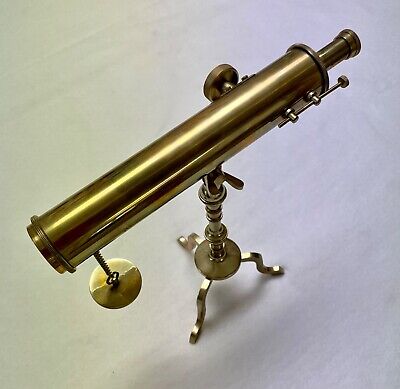The image depicts a vintage-style, brass tabletop telescope placed on a white table, captured from a bird's-eye view. The telescope, finished in a dull, dark gold hue, rests on a three-legged holder and includes an adjustment bar for raising or lowering the viewing angle. It features a cap hanging off the end by a chain and an adjustment button. The eyepiece is located at the smaller end on the top right of the image. The background is a pale gray, enhancing the antique aesthetic of this compact telescope, which is oriented with the eyepiece facing rightward.